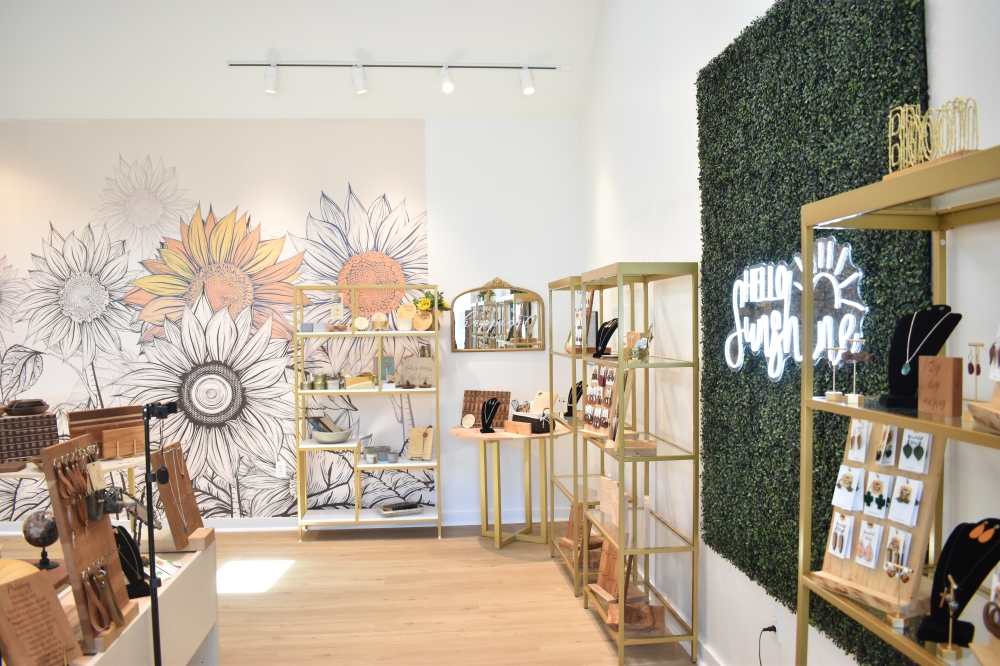The photograph depicts the inviting interior of a boutique jewelry store, characterized by its high ceilings and well-lit ambiance. Upon entering, one is greeted by gold-colored open shelves displaying various jewelry items, including earrings and necklaces, primarily arranged on black display holders. The store has white walls and wood flooring, creating a warm and airy atmosphere. 

To the right, a striking feature is a textured faux grass wall adorned with a white neon sign that reads "Hello Sunshine," accompanied by a stylized sun outline. This greenery adds a refreshing touch to the otherwise modern decor. The opposite side of the room showcases a large wall mural of sunflowers, predominantly in black and white, with a couple of the flowers highlighted in vibrant orange and yellow hues, adding a splash of color that catches the eye. This artistic display could signify either an unfinished piece or a deliberate design choice by the artist.

Additional furniture includes a table partially visible on the left, holding wooden display boards with more merchandise. The well-lit space is enhanced by studio lights hanging from the white ceiling, ensuring all areas are bright and welcoming. Overall, this store presents a modern yet cozy shopping experience, accentuated by its thoughtful decor and detailed displays.